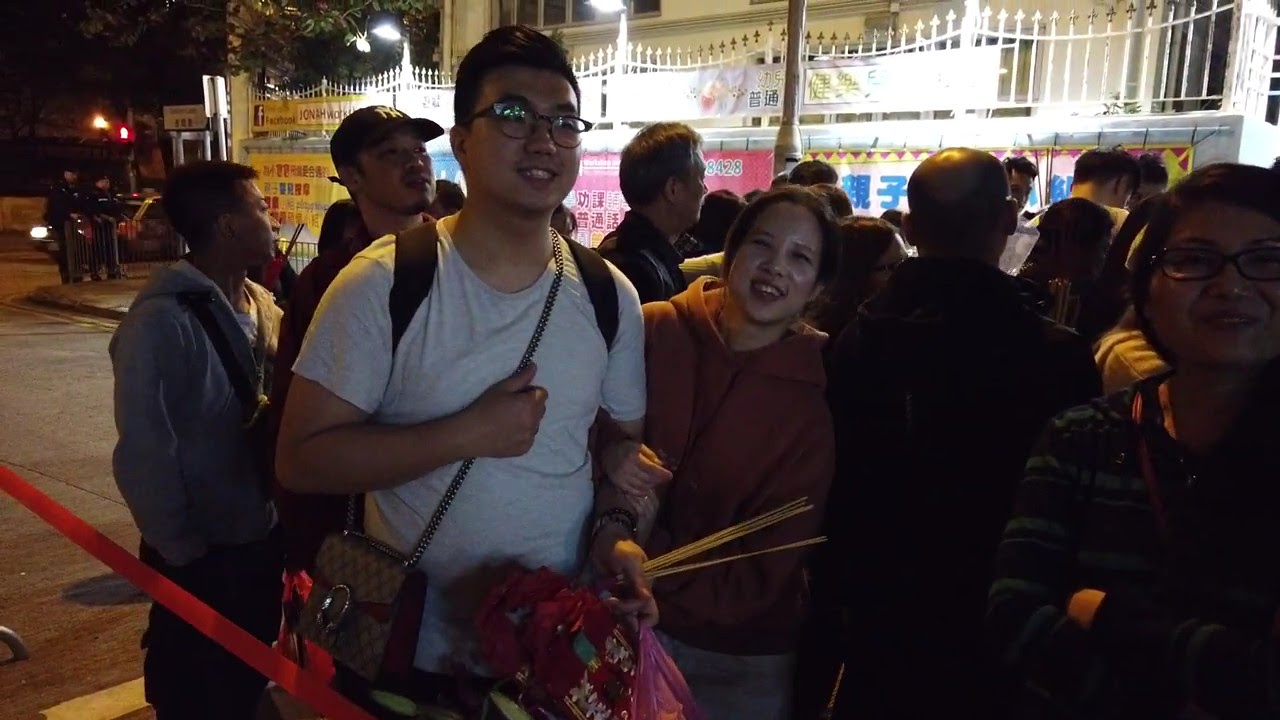In this nighttime scene at a bustling fair or carnival, a diverse crowd, primarily of young adults, is gathered, creating an atmosphere of lively anticipation, possibly waiting in line for a show. The vibrant background includes food booths adorned with Chinese or Japanese text, adding an international flair to the setting. 

Dominating the foreground is a man in his twenties, wearing black-framed glasses and a white short-sleeved t-shirt. Strapped over his shoulders is a black backpack, and he clutches a pink, flowery item with stick-like embellishments in his left hand. The man also carries a purse or similar accessory, suggesting a fashionable or practical nuance. Beside him, a girl in a brownish hoodie grasps his elbow, while to the right, another girl in a striped shirt is visible.

Notably, a red ribbon or tape runs diagonally from the middle bottom to the side middle of the image, perhaps marking an area off-limits to the crowd. Everyone seems engaged and joyous, highlighting the event's communal and festive aura.